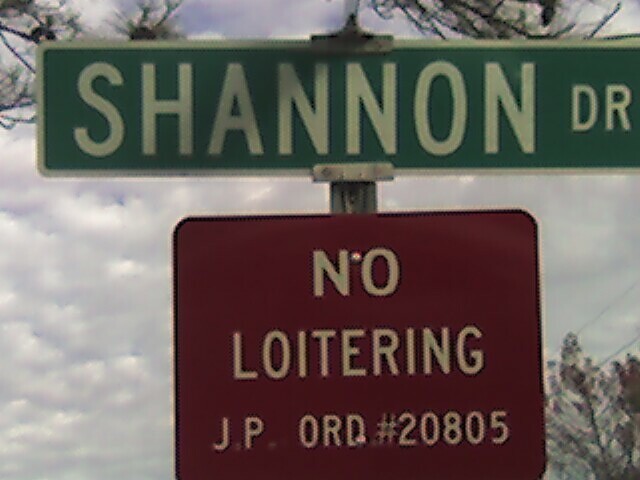The image depicts a pair of signs mounted on a silver pole. At the top is a green street sign with a white border that reads "Shannon DR," the abbreviation standing for Shannon Drive. Directly beneath it, there's a red rectangular sign with rounded corners, displaying the message "No Loitering, J.P.ORD #20805" in white lettering. The background showcases a cloudy sky with various shades of white and gray, interspersed with patches of blue. Surrounding the signs are tree branches, visible in the top left and right corners of the image, along with some power lines near the trees on the right side, all contributing to a detailed, overcast ambiance.